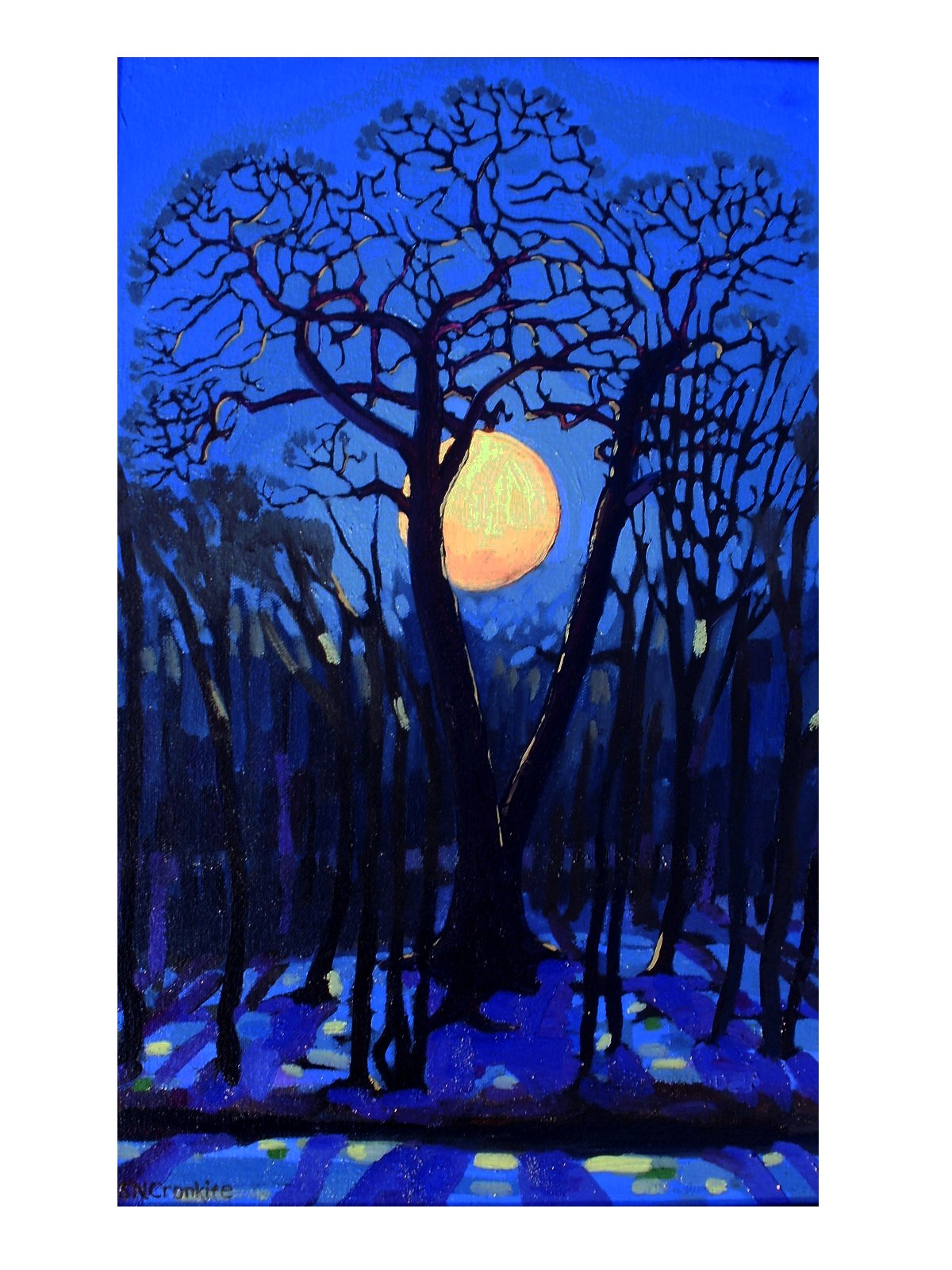The image is a tall, classical surrealism painting of a forest at night, dominated by dark blues and blacks with a hint of surrealistic artistry. At the forefront, a variety of trees stand bare, with their branches resembling intricate capillaries or ventricles. The largest tree, centrally located, features a striking Y- or V-shaped form that stretches skyward. Within the open arms of this centerpiece tree, a partially obscured, full moon glows with an orange-y yellow hue, casting subtle shades of blue, gray, and black across the scene. The ground below hints at a snowy covering, reflecting the moonlight in varying shades. All surrounding trees lean away from the grand central tree, bending towards the left and right edges of the painting, framing the moon perfectly in the forest's mystique. This composition suggests a serene, yet slightly eerie, winter night in a dense wooded area.